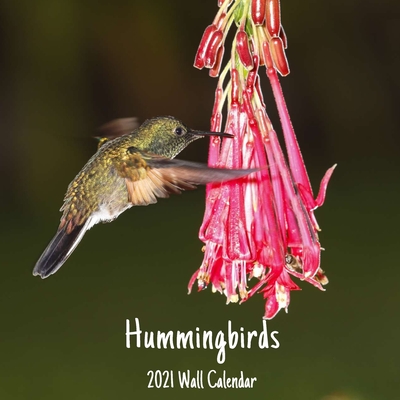The image displays the front cover of a "Hummingbirds 2021 Wall Calendar". The background is an out-of-focus dark green, providing a muted backdrop that highlights the central elements. Towards the right-hand side center, there's a prominent pink flower hanging downward, reminiscent of a fuchsia flower, with many cascading petals. To the left of the flower hovers a tiny hummingbird in mid-flight, its greenish-brown feathers with touches of yellow and gray visibly fluttering, while its beak is poised to drink from the flower. The hummingbird sports a dark gray tail. At the bottom of the image, in clear white text, the title "Hummingbirds" is boldly displayed, followed by “2021 Wall Calendar”. There are no other elements such as additional animals, people, buildings, or vehicles, ensuring the focus remains solely on the vibrant interaction between the flower and the hummingbird.